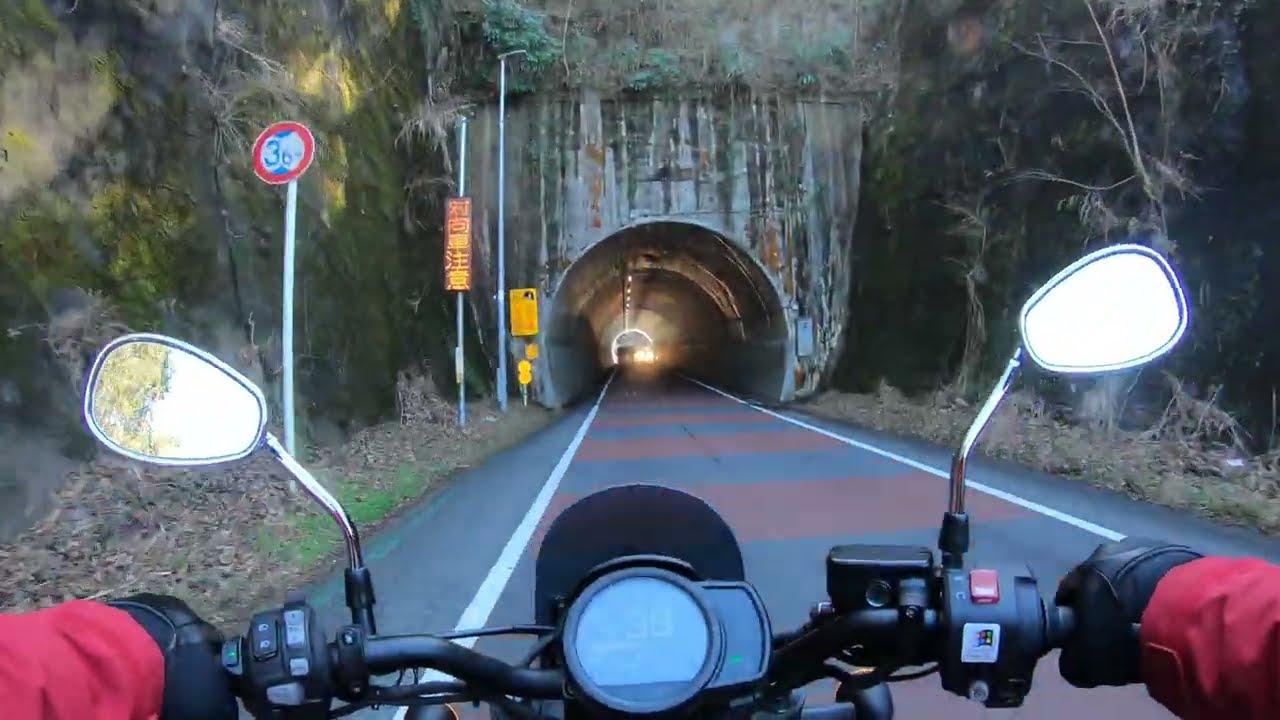The image captures the point of view from a motorcyclist approaching a tunnel under a mountain during daylight. The bottom of the image features two chrome side mirrors and hands in black gloves with red sleeves gripping the handlebars, highlighting the rider in motion. The dark gray asphalt road has a distinctive horizontal brown and gray pattern, adorned with red diagonal lines and white traffic markings. To the left, a speed sign marked "36" stands near a rocky formation with sparse grass. On the right side, dry trees frame the path. The tunnel entrance, constructed with concrete, glows with a bright yellow light, suggesting illumination from within. Overhead, dead foliage clings to the rocky landscape above the tunnel entrance.